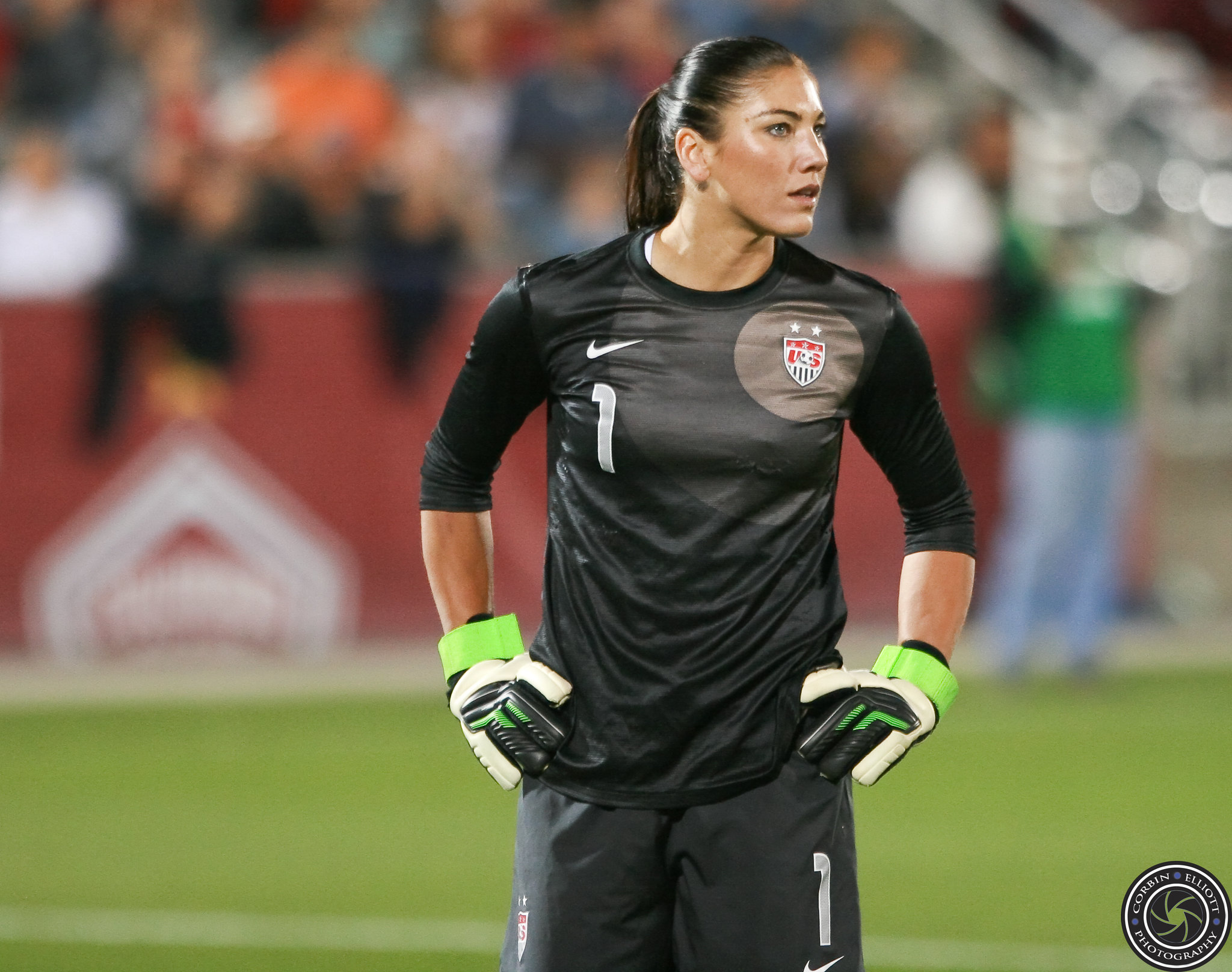This image captures a female goalkeeper on a football pitch, where the entire background is artistically blurred, emphasizing the colors red, green, blue, black, orange, and white. The goalie, positioned prominently in the foreground, has her dark hair pulled back and is showcased from the side view, revealing her blue eyes. She is dressed in a black sports uniform with a white number one on both her jersey and shorts, complemented by a white Nike emblem. Her goalkeeping gloves are padded with a dynamic mix of red, black, green, and white. She appears to be looking towards the right side of the frame, away from the camera. At the bottom of the image, there is a logo with text that reads "Corbyn Elliott's Photography." In the blurred background, hints of grass, a wall, and spectators in the stands can be discerned, adding context to the sporting event.